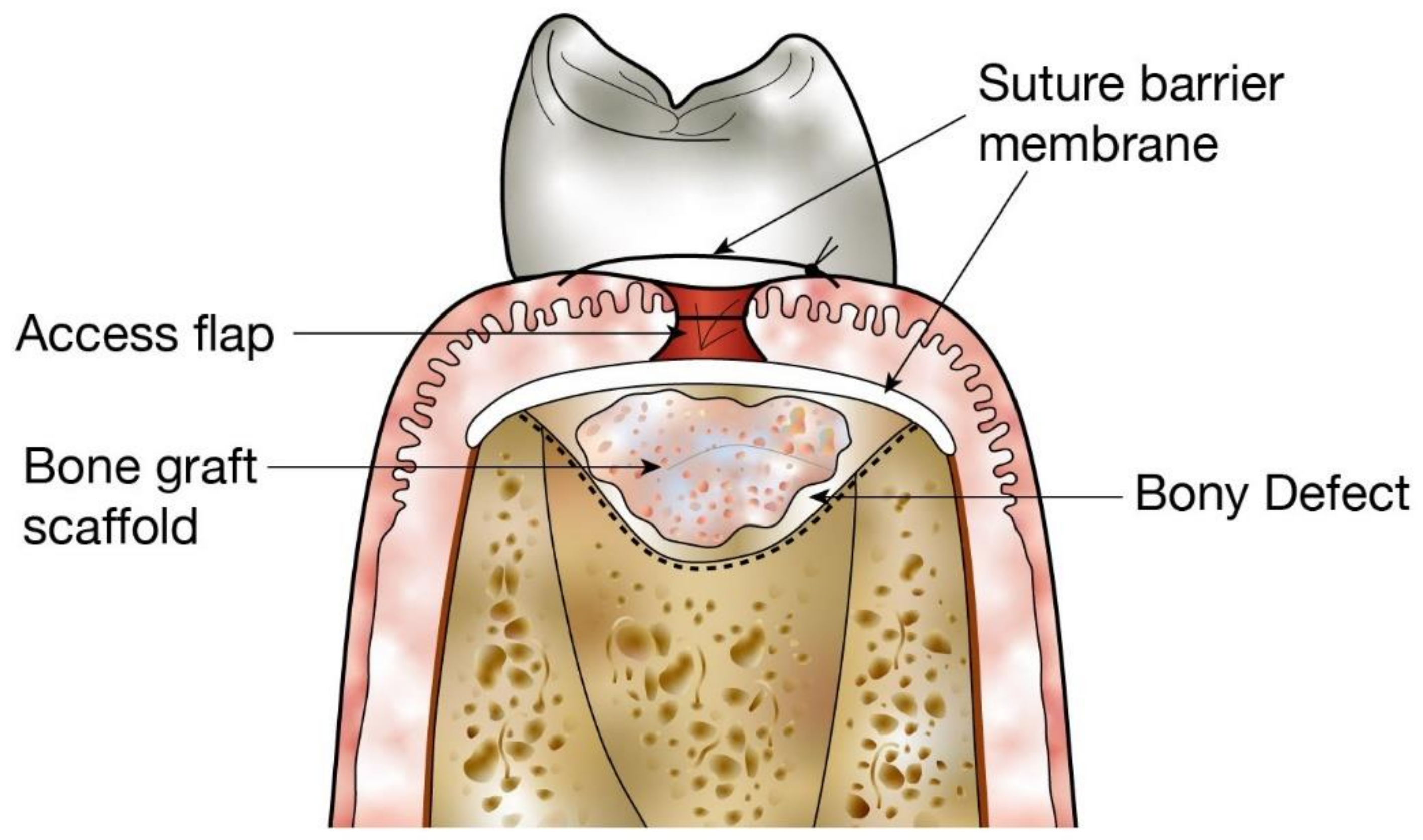This detailed illustration depicts a cross-section of a tooth within the gums, set against a white background. The upper portion is a tooth, which appears grayish and is illustrated in a detailed manner. Below the tooth, the image transitions into a pink U-shaped gum area. The interior of the gums reveals a complex view of the bone structure involved in a dental operation. Various parts are labeled with arrows in a clockwise fashion: starting from the upper right, they indicate "suture barrier membrane," "access flap," "bone graft scaffold," and "bony defect." The scaffold and defect areas inside the gums show a mix of peach, tan, and brown colors, visually representing the intricate details of the dental process.